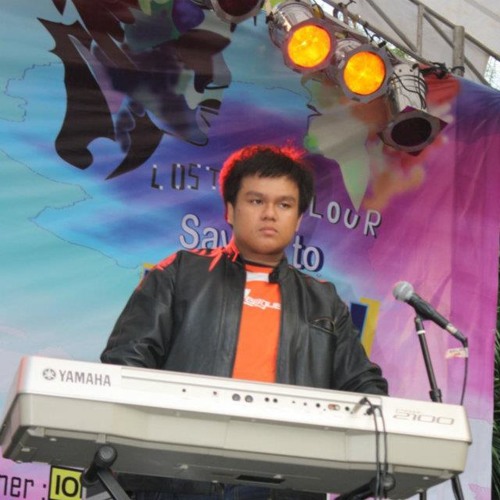A young Filipino boy, with slightly poofy black hair and a chubby build, is performing on stage. He is standing behind a gray Yamaha keyboard, model 2100, mounted on a black stand. He is dressed in a black leather jacket over an orange shirt, and a black microphone is positioned next to the keyboard. His expression is serious as he gazes into the audience. Behind him, a large banner features abstract faces and the text "LOST" to the left of his head, and "LOUR" to the right, with other partially obscured letters. The banner's background transitions from pink on the right to blue on the left. Above the boy, stage lights emit a yellow glow, adding to the vibrant hues of the backdrop. The scene suggests he might be part of a band, potentially singing while playing the keyboard.